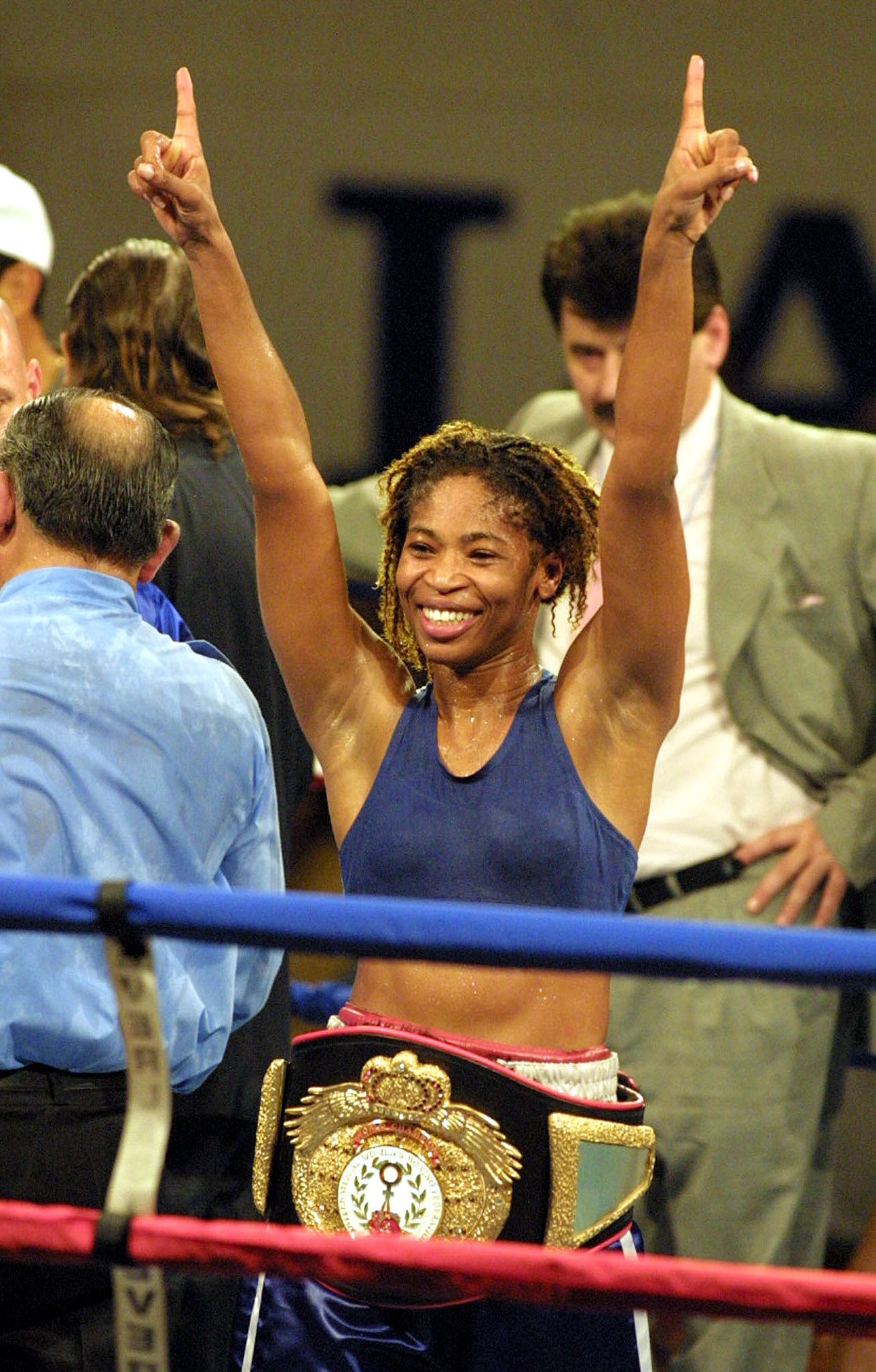This vibrant color photo captures a triumphant moment of an African-American woman celebrating her victory in a boxing match. With both hands raised high and her index fingers pointing skyward, she exudes joy, grinning widely while looking off to the side. She is dressed in a coordinated navy blue sports bra and boxing shorts, complemented by a striking championship belt around her waist. The belt features an elaborate gold ornament design with wings across the top, a central white circle adorned with olive leaf branches, and is bejeweled with red rhinestones, making it shimmer as a testament to her achievement.

The image is framed through the ropes of the boxing ring, with a blue and red top rope visible. In the background, a man in a green suit with olive pants and a white shirt looks on proudly, positioned directly behind her. To her right stands another man, balding and sweaty, dressed in a blue shirt, further adding to the celebratory atmosphere. The ring ropes and the bustling figures in the background suggest a lively and energetic post-match scene, capturing the essence of her hard-fought victory.